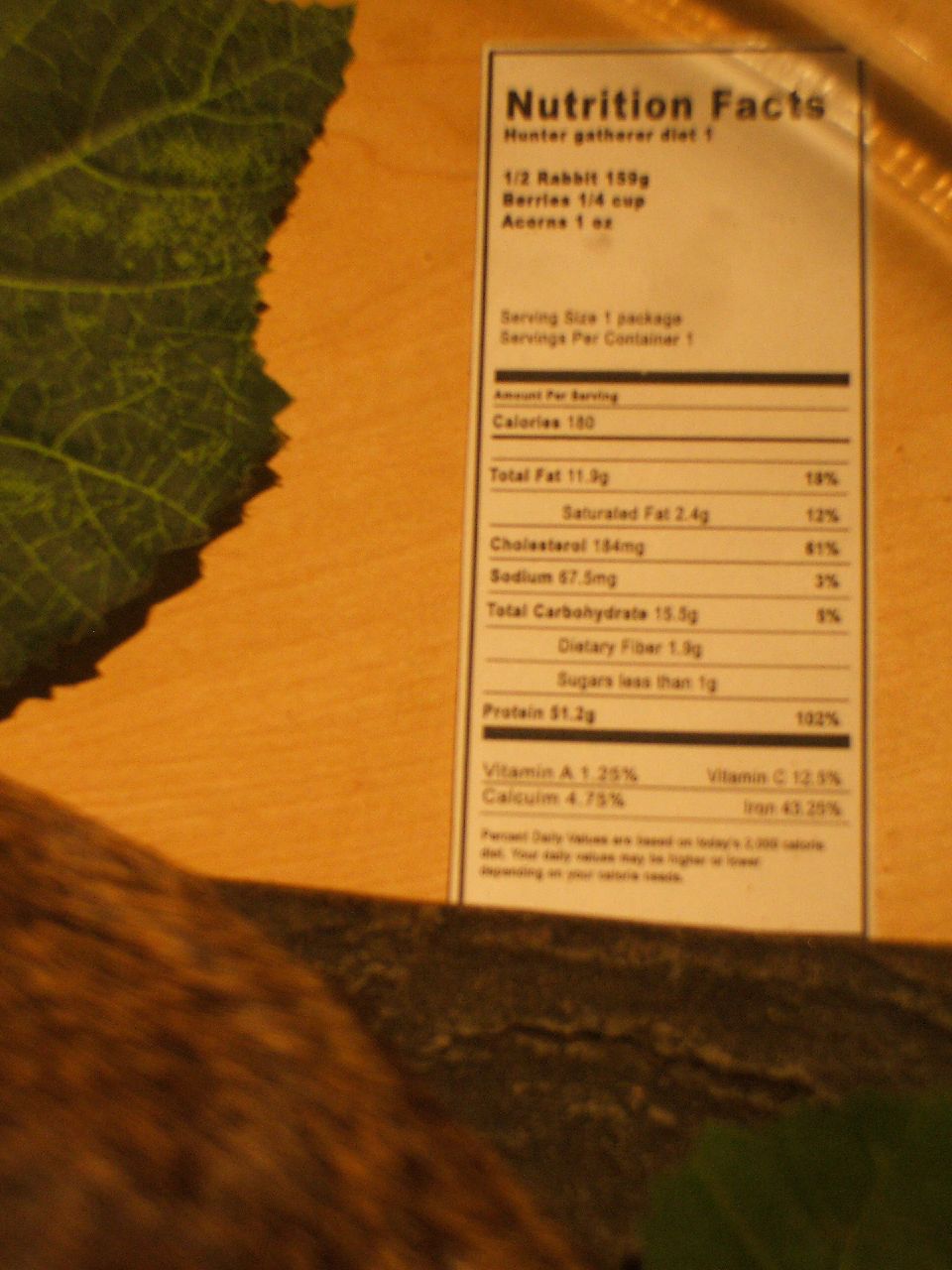The image displays a nutritional information label set against an orange backdrop, which resembles a table or possibly the packaging itself adorned with tree bark imagery. Green leaves are partially visible on both the left and lower right sides. The label is blurred but identified as listing the nutritional facts for a meal described as "Hunter-Gatherer District 1." The ingredients include half a rabbit (159 grams), a quarter cup of berries, and one ounce of acorns. The serving size is indicated for one person, with a total of 180 calories. The label details the amounts of fat, cholesterol, sodium, carbohydrates, and protein in the meal, suggesting it is designed for a camping experience or a diet mimicking hunter-gatherer traditions.